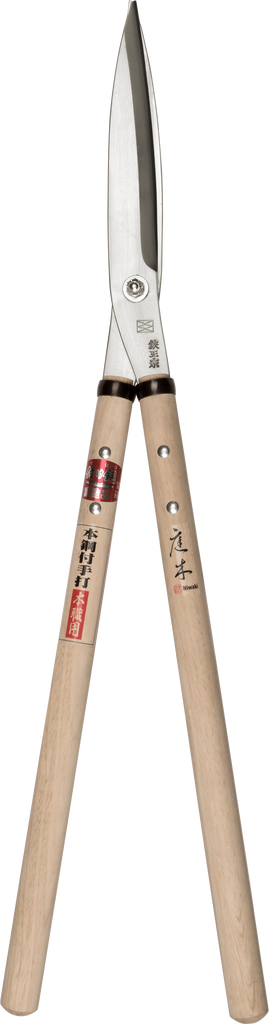This close-up image showcases a pair of large, silver garden shears with a distinct Japanese aesthetic, designed for trimming bushes. The shears feature long, thin handles made from light-colored wood, adorned with several pieces of Japanese writing. The left handle displays Japanese characters near the top, followed by a red rectangle with additional Japanese text. Similarly, the right handle has more Japanese writing, with two characters or symbols near the top, a small red symbol below, and a tiny section of English text that requires a magnifying glass to read. Both handles are secured by silver bolts at the top. The tool itself comprises two sharp silver blades, joined at the center by a screw, with a black ring just above the handles. The image background is plain white, which helps to highlight the intricate details and markings on the shears.